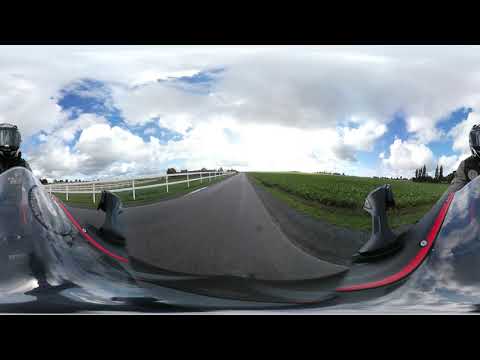The image is a panoramic, point-of-view shot of a motorcyclist riding a sleek, glossy black motorcycle down a dark asphalt country road that lacks lane markers. The motorcyclist is wearing a black jacket with grey sleeves, featuring a grey circular logo on the front, and a black helmet with a dark reflective visor pulled down. Due to the 360-degree imaging, the image appears split, causing the rider to be visible on both the right and left edges of the photograph.

Ahead of the motorcyclist, the open road is welcoming with no other vehicles in sight. On the left side of the road, there is a white wooden rail fence with well-spaced posts, behind which stretches a flat green grassland field. On the right side, there's a gravelly shoulder leading to what seems to be a field of green leafy crops or shrubs. In the background, the sky is light blue, filled with thick white clouds, and the sun is positioned toward the center of the image, casting a serene light over the entire scene. In the upper right corner, some trees are visible, adding to the rural charm of the landscape.